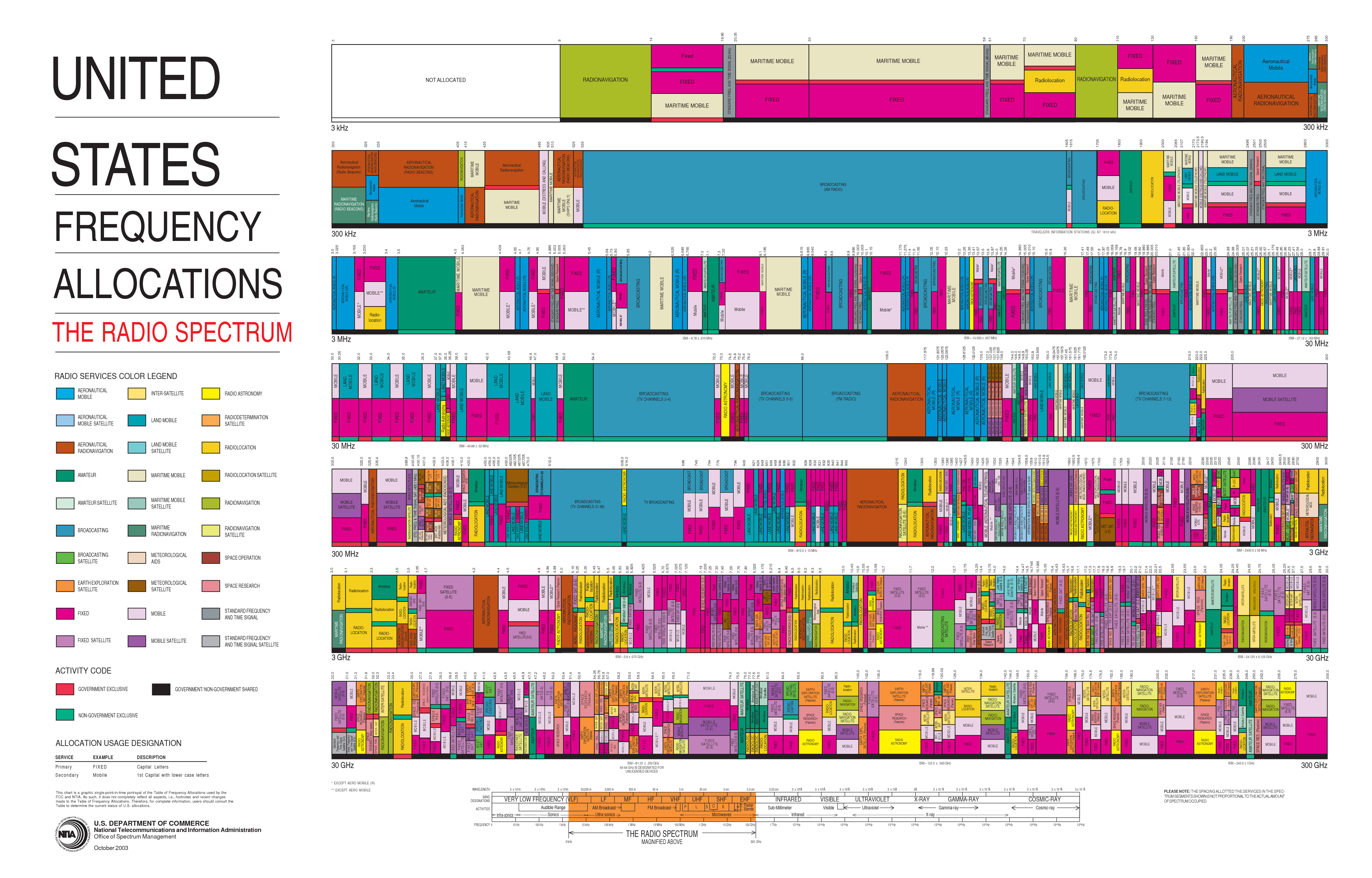This image captures a detailed poster titled "United States Frequency Allocations" located in the upper-left corner, with a subtitle in red reading "The Radio Spectrum" just below it. The poster exhibits a comprehensive visual representation of the radio frequency spectrum, employing a color-coded system to categorize various radio services. A legend termed "Radio Services Color Legend" on the poster acts as a key, explaining the significance of each color. The spectrum chart features myriad colors including green, purple, pink, yellow, white, black, and gray, each symbolizing distinct radio services. The chart is structured with rectangles of varying sizes and orientations—some are long, some short, some vertical, and others horizontal—indicating different frequency allocations. Toward the bottom, an orange-highlighted segment labeled "Radio Spectrum Magnified Above" provides an enlarged, more detailed view of a specific section of the spectrum. This intricate and colorful chart serves as a valuable reference tool for understanding the allocation of radio frequencies in the United States.